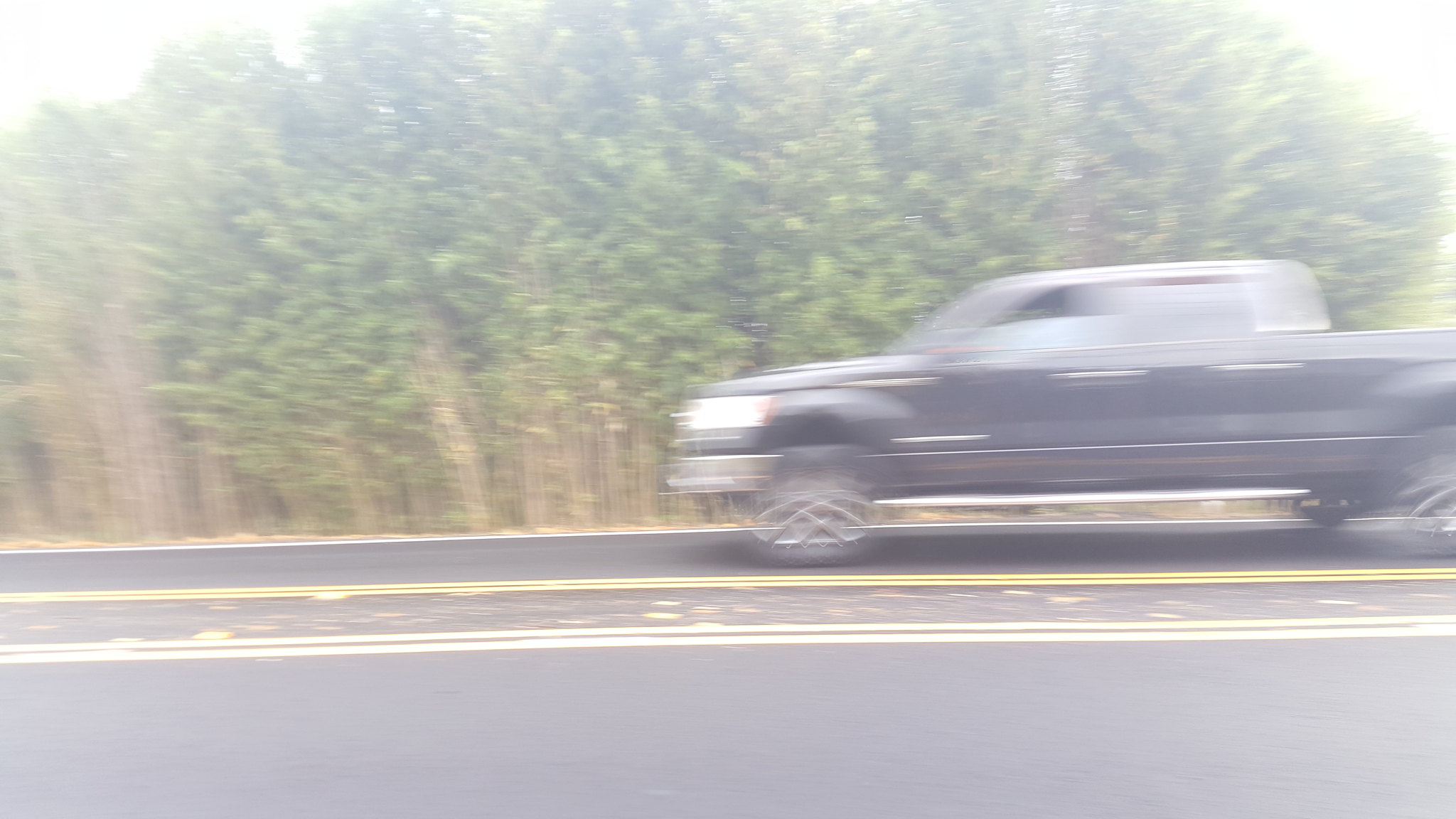A large, dark gray pickup truck speeds down a newly paved, two-lane road, evidenced by its slight blur in the image. The road, featuring a vivid double yellow line and a narrow center lane, appears freshly surfaced with deep black asphalt. Surrounding the scene is a backdrop of tall, dense trees, suggesting the truck is traversing through a wooded area. Despite the road's seemingly busy nature, the truck is the sole vehicle captured in this image, underlining its prominence. The truck's spacious cargo bed indicates its capability for hauling substantial loads.